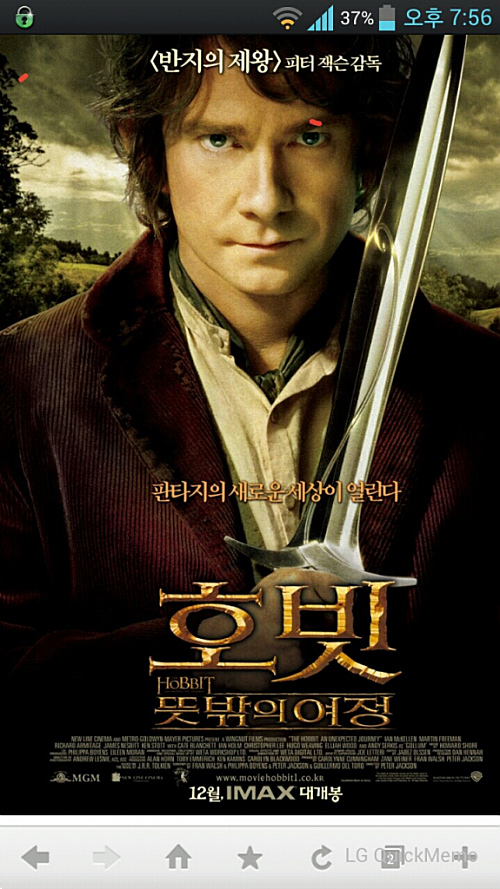This is a detailed movie poster for "The Hobbit," showcasing a computer-generated, hyper-realistic image of a young white man with long brown hair and greenish-blue eyes, standing in a serious, contemplative pose. He is dressed in a dark brown sport jacket, a white shirt, and a green scarf, holding a silver sword against his shoulder. The background features vivid clouds with sunlight streaming through and some trees, adding a dramatic effect. The poster is primarily in an Asian language, presumably Chinese or Japanese, with the only English words being "IMAX" and "Hobbit." The poster appears to be a screenshot from a cell phone, evident from the top bar displaying a Wi-Fi signal, cell reception, a battery at 37%, and the time at 7:56. The bottom of the screenshot includes navigation icons and some unintelligible letters and symbols, suggesting it might be part of a screen dump.